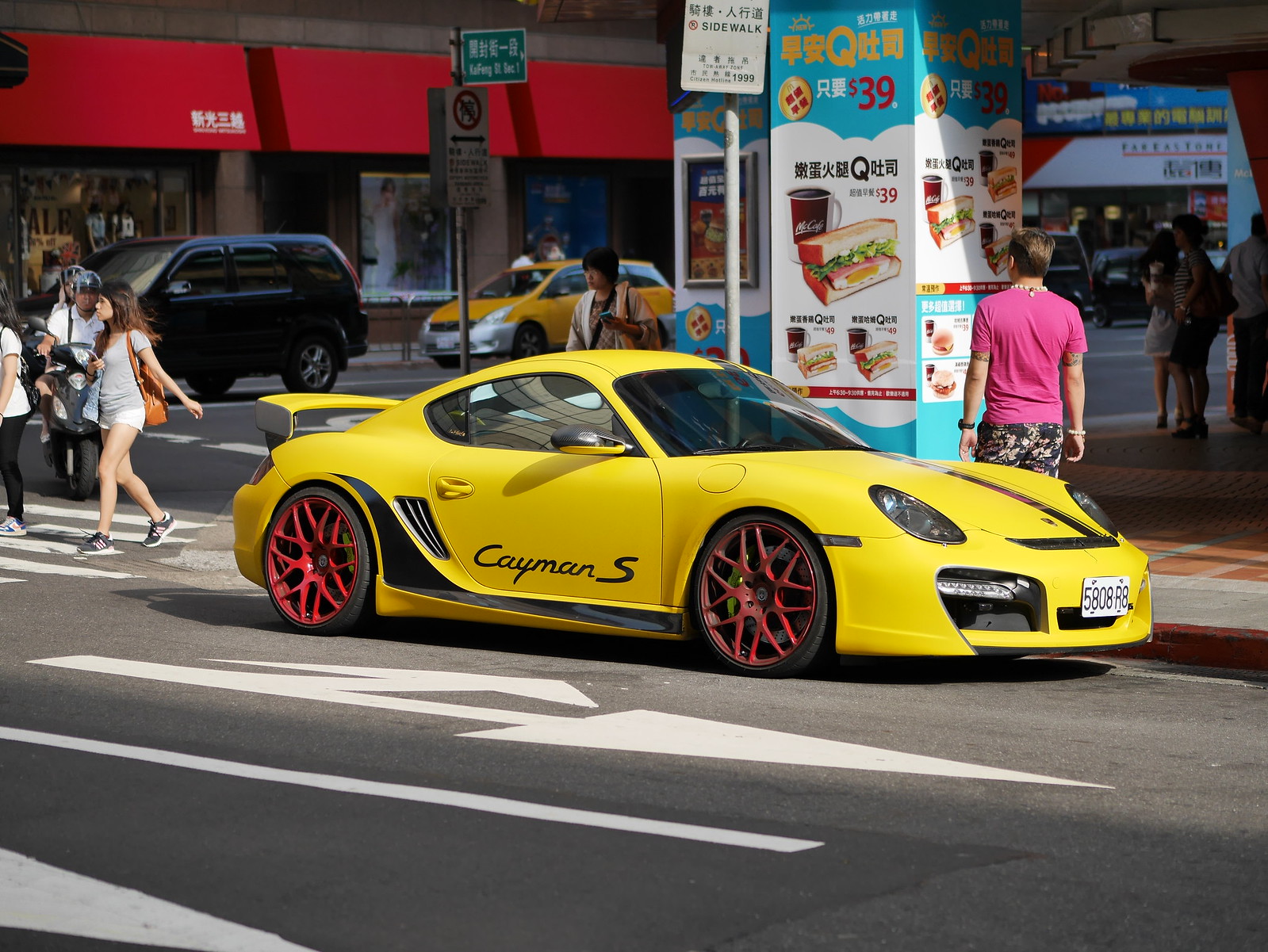In this vibrant urban street scene, a striking yellow Porsche Cayman S, adorned with a black stripe down its hood and red six-spoke rims, is prominently parked by the curb. The sleek sports car features a white license plate displaying the numbers 5808 R8 and a distinctive yellow rear spoiler. The bustling backdrop suggests an Asian city, amplified by a kiosk selling sandwiches with Chinese or Japanese writing, advertising a fast food combo with a sandwich and a Dr. Pepper. Around the car, well-dressed pedestrians, including a young woman in a light white t-shirt, short shorts, and tan trainers carrying a shoulder bag, navigate the lively street. Several taxis and diverse vehicles, including a motorbike with a blue helmet and a dark van, punctuate the scene, while numerous small businesses, eateries, and a clothing store enhance the urban ambiance.